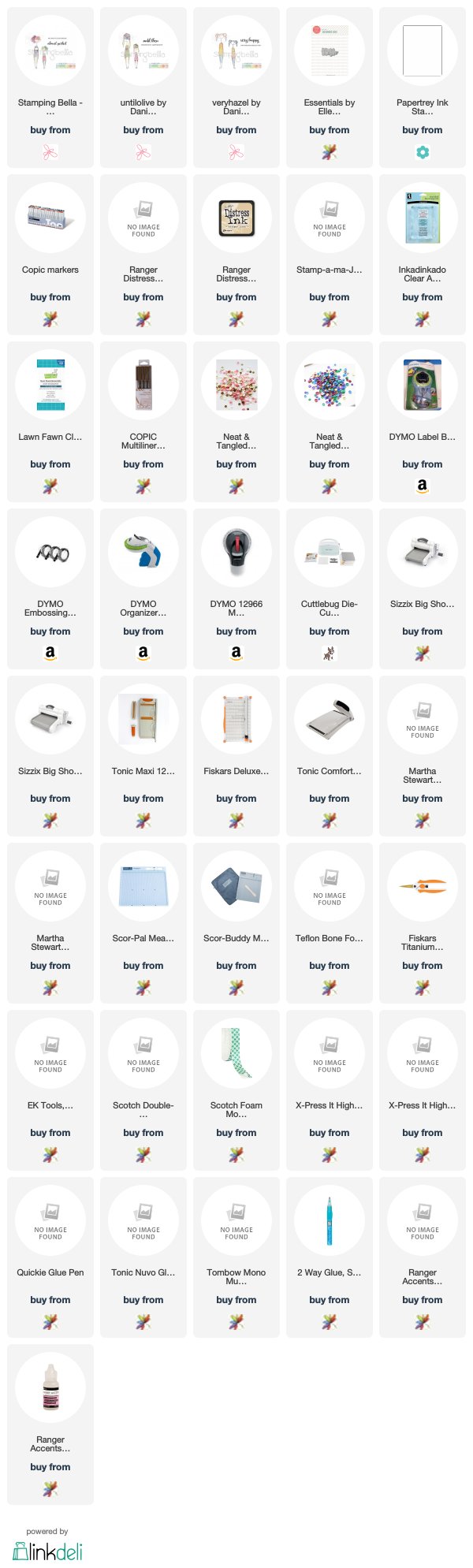The image depicts a grid layout featuring multiple small boxes, each containing different items. The grid consists of nine rows, with the first eight rows displaying five items each and the last row featuring just one item. Each box includes a title and a "Buy From" link. The topmost item appears under the brand name "Stamping Bella," followed by a "Buy From" option beneath it. 

The visual elements indicate that some items are available on Amazon, while others come from various other companies. Below the final row, there is a note indicating that the display is powered by Ink, specifically through Link Deli. The word "Link" is presented in black font, whereas "Deli" appears in a greenish-aqua font. Additionally, there is a logo featuring a shopping bag positioned to the left of the text. The overall layout suggests a neatly organized list of products, each with a corresponding purchase link for ease of access.